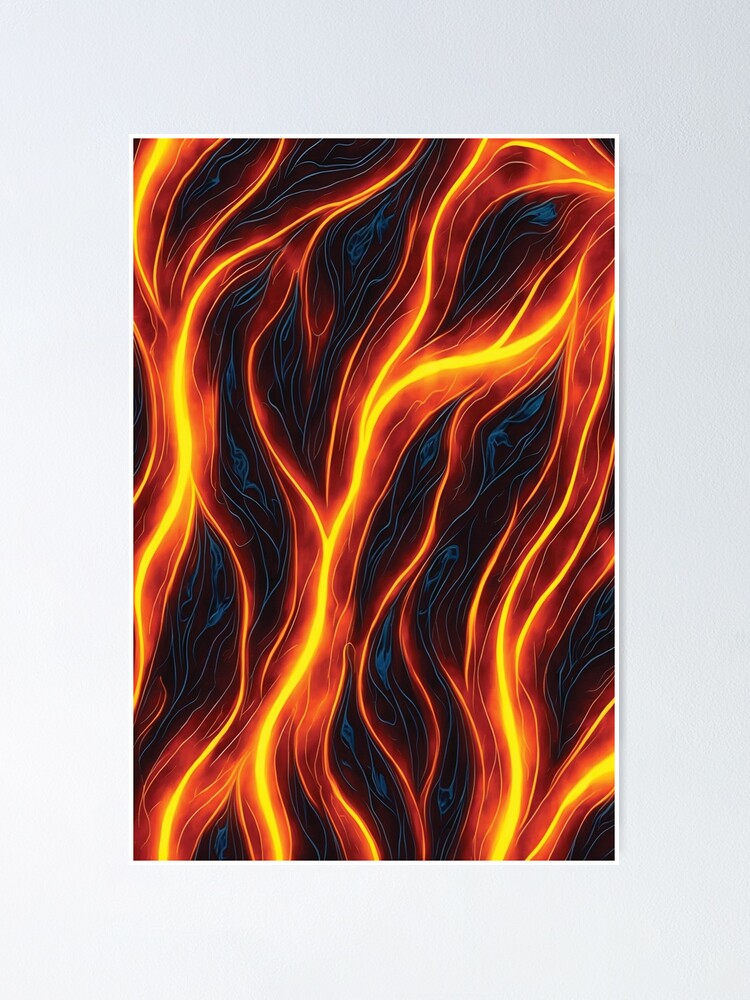The image is an abstract art piece primarily depicting flames. It is oriented vertically, framed by a narrow white strip on light gray edges. The background is predominantly black, interspersed with subtle, barely discernible blue lines that thread through the composition. The central focus of the piece is an array of vibrant, wavy lines mimicking fire, dominated by bright yellow and rich orange hues, highlighted by thinner, more intense orange-yellow strokes. The flames appear to branch out with varying thickness, creating a dynamic, vessel-like pattern reminiscent of fire. The overall effect is a vivid portrayal of flames, emphasizing their fluid, intricate motion set against a dark backdrop.